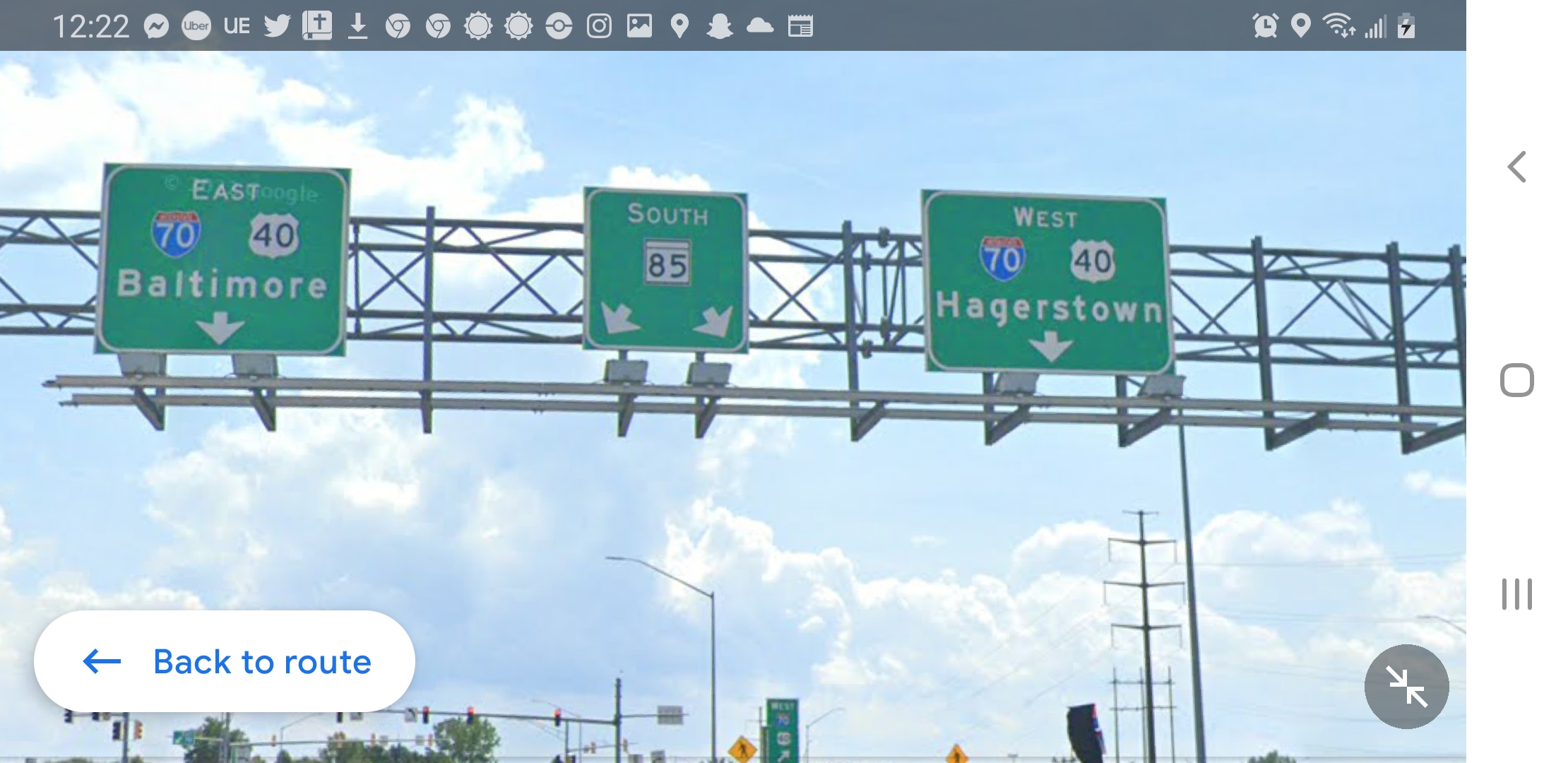This colour image, possibly captured from a computer or tablet screen, prominently features a set of street signs against a backdrop of a blue sky with scattered clouds. At the top of the screen, a black bar displays various white icons, including a clock on the left, multiple status icons in the center, and a wireless signal indicator and battery icon on the right, suggesting the image might be viewed on a digital device.

Dominating the foreground, there is a large metallic pole stretching horizontally, supporting three square green signs with white text. 

- The leftmost sign reads "East 70 40 Baltimore" with a downward arrow, and also features a circular icon with the number "70" inside it.
- The middle sign displays "South 85" accompanied by a circular icon with the number "70" and has arrows pointing towards the bottom corners.
- The rightmost sign states "West 70 40 Hagerstown" with a downward arrow.

In the distance, more signs and what appears to be a streetlight are visible. Trees are seen on either side, providing a sense of depth and location. 

In the bottom left-hand corner, there is a blue rectangular button with curved edges labeled "back to route" and an arrow pointing to the left. The bottom right-hand side of the image includes a grey circular icon with two white arrows converging at the center.

The details provided give the viewer a clear understanding of the location and layout of the street signs and surrounding elements in the image.